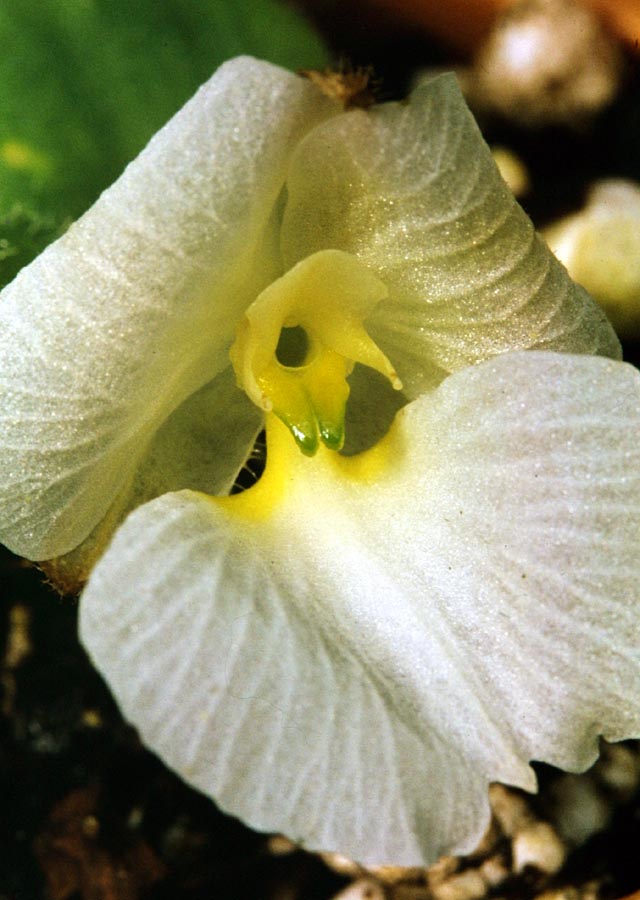This close-up photo showcases an intriguing orchid with a highly detailed structure. The orchid boasts three petals: one at the center bottom that is wide, and two at the top corners, which are folded and curled. These petals are a mix of white and translucent hues, with visible veins running through them. The middle part of the flower features a distinctive hole surrounded by a sparkly, crystalline texture. There is a flare at the top center, and two greenish spikes that descend from the bottom. A touch of yellow from the center subtly blends into the white petals. In the upper left corner, a green leaf extends from the flower, while the backdrop of the image is dark and blurry, resembling dirt. The fascinatingly unique and translucent nature of the petals, coupled with the sparkling details and the unfolding leaves, makes this orchid a truly captivating subject.